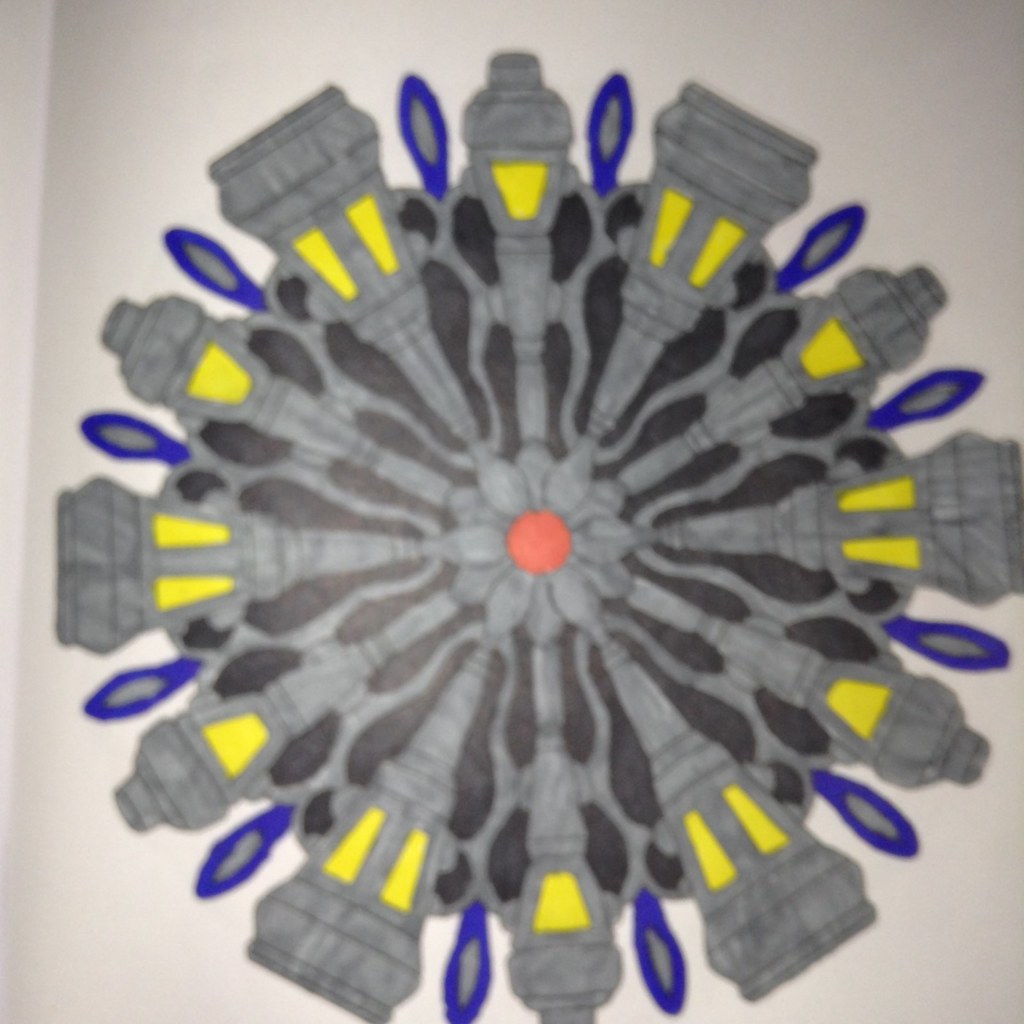This artwork presents a visually complex, flower-like motif set against a light gray background. The central part of the "flower" is peach-colored, surrounded by a ring of small gray petals. Extending from this center are multiple segments that form the larger structure. These segments are narrow at the base, gradually widening towards the top, which features two yellow slits. Additionally, between each of these dual-slitted segments, there's another segment capped with a single yellow slit. Adorning the intervals between these segments are bright blue petals with gray centers, further enhancing the intricate design. Black borders meticulously outline the elements within the composition, contributing to the striking contrast between the black, gray, yellow, and blue hues. The overall appearance resembles a stylized flower, although the petals have a distinctly geometric, boxed-off appearance.